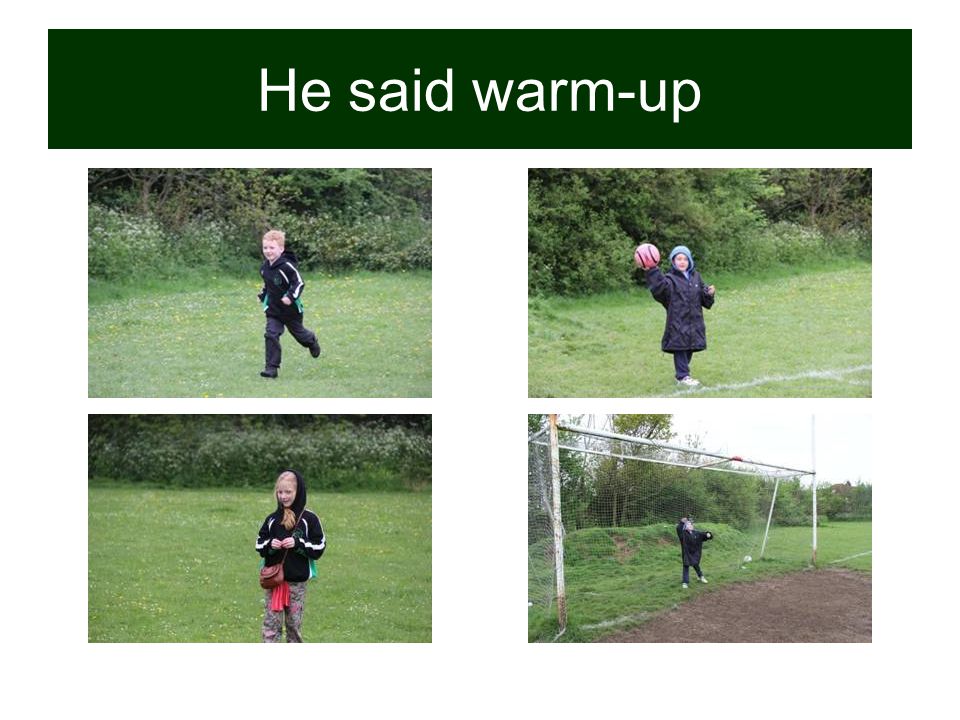The image is a collage of four photographs depicting children playing outdoors, arranged in two rows and two columns against a white background. At the top of the image, there's a green rectangular banner with white text that reads, "He Said Warm Up." Each photograph captures a different scene in the same grassy, tree-lined area, suggesting they might be warming up before a game or activity. 

In the upper left photograph, a little boy with short, sandy blonde hair is seen running on the grass. He wears a dark jogging suit with a stripe down the arm. The upper right photograph shows a girl in a long black jacket and pants standing in the same grassy area, holding up a basketball with her right hand. She has a blue hood on. 

The lower left photograph presents another girl with blonde hair, wearing a black jacket with a stripe down the arm and a pinkish purse around her neck. She is standing with her hood up and something pink hanging down in front of her pants. The lower right photograph features a child standing in front of a rusted soccer goal net, partially obscured and reaching for something. The various colors in the scene are predominantly green for the grass and trees, with accents of black, pink, red, and blue in the children's clothing. The overall setting appears to be a park in the middle of the day, indicated by the natural light and outdoor environment. The children are dressed in heavy jackets, suggesting that it might be a cold day.